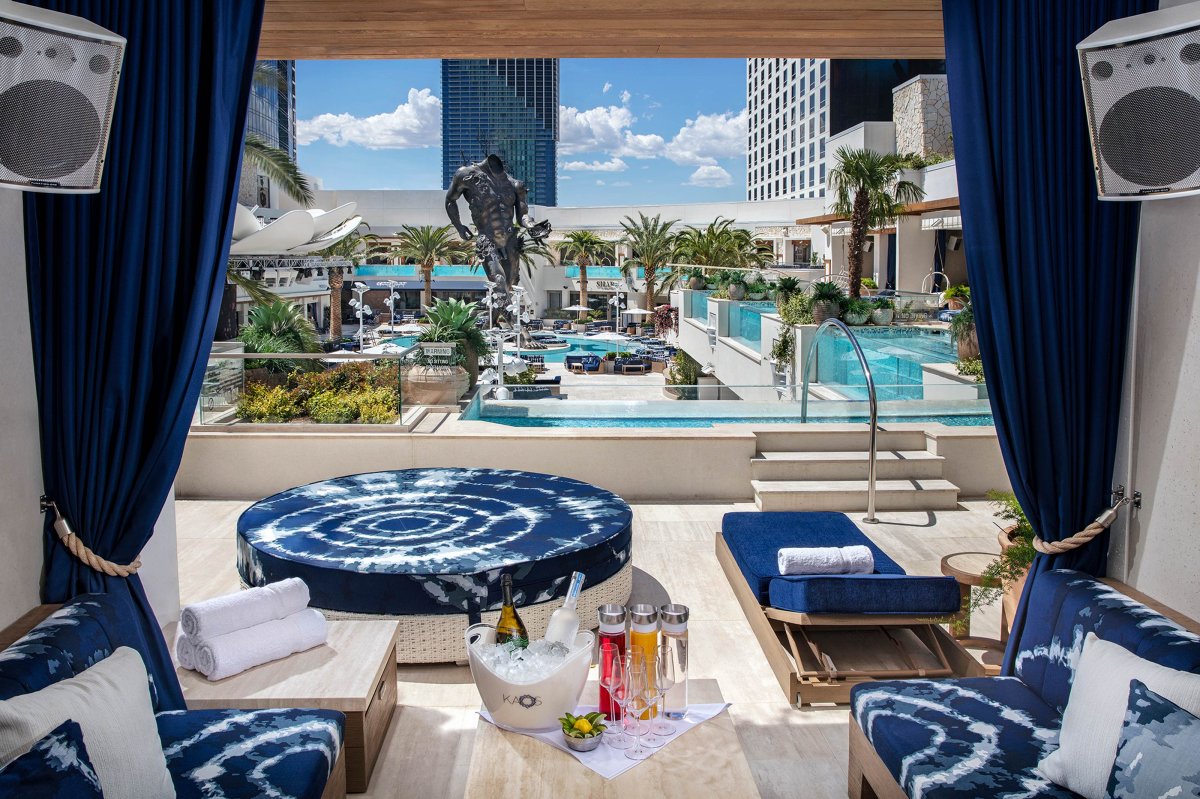The photograph, taken from the perspective of a luxurious cabana or high-end hotel room at the Palms Casino Resort in Las Vegas, Nevada, offers a detailed view of a lavish pool and cabana area. The shot is framed by blue curtains with gold tiebacks that hang from wooden rafters. The stone patio outside features dark blue furnishings with white tie-dye patterns, including a large round couch, a chaise lounge on a wooden base, and several other sofas. There is an ottoman table and end tables with towels rolled into a pyramid and an ice bucket with champagne and various drinks. Inside, matching tie-dye styled furnishings and an ice bucket are visible beneath the cabana's speakers, adding to the luxe atmosphere. The outdoor pool area is surrounded by tall palm trees and numerous floors of the white building, extending out of the image up to the top right, indicating many floors. At the center of the pool area stands a tall, grey statue of a headless male figure, and the poolside is dotted with chairs for guests, set against the backdrop of glass walls and the blue sky.